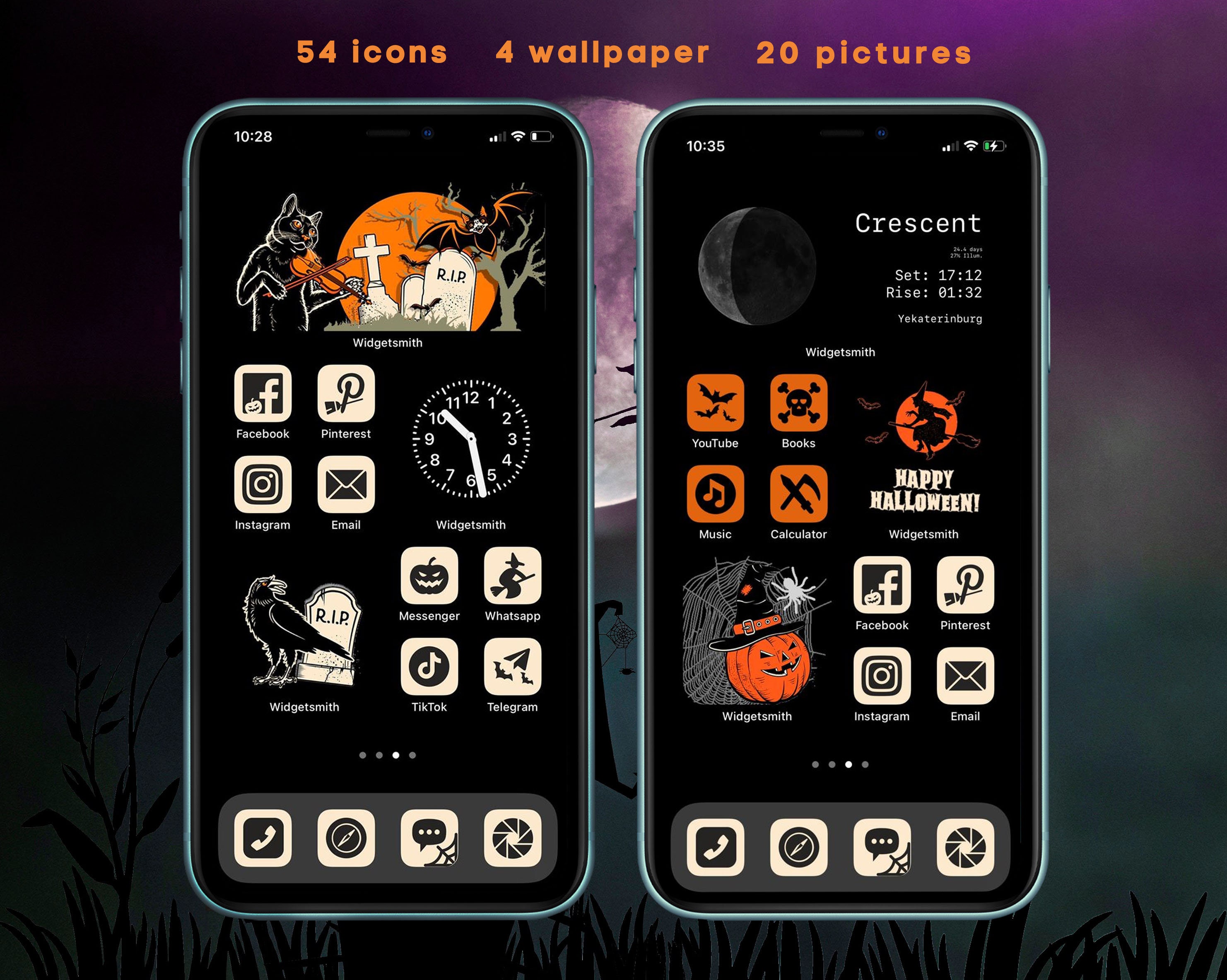In this image, we see two mobile devices side by side, each displaying their home screens. The first device, positioned on the left, displays the time as 10:28. It shows network signal strength just shy of full bars and a full-strength Wi-Fi signal. The home screen includes 54 icons spread across different folders and apps, with 4 wallpaper options visible in the background, along with 20 picture thumbnails.

The second device, positioned on the right, shows the time as 10:35. Its network signal strength is also just short of full bars, and it has a strong Wi-Fi signal indicated by full bars. The battery level indicator on this device shows that it is currently charging. The home screens on both devices feature a variety of commonly used applications, including Facebook, Pinterest, email, Instagram, Messenger, WhatsApp, Telegram, TikTok, music player, YouTube, books app, calculator, messaging app, camera, phone dialer, and Safari browser.

Overall, the image provides a comprehensive view of the home screens, showing various app icons and system indicators, reflecting the activity and connectivity of both devices at the annotated times.